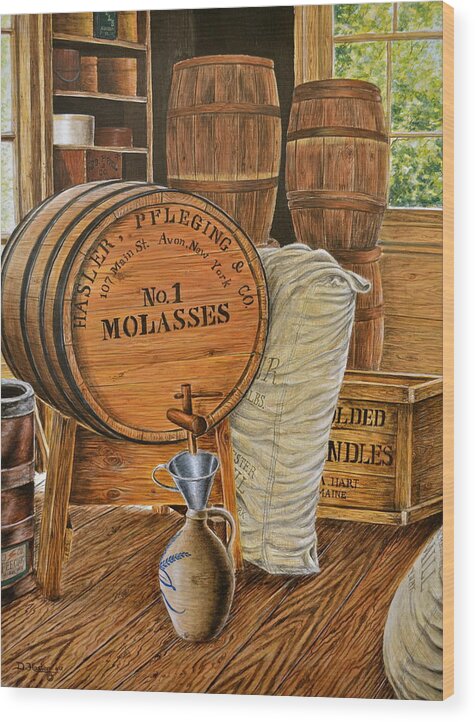The drawing is set inside an old-fashioned barn or general store where molasses is produced. Dominating the scene is a large barrel labeled "Number One Molasses" from Hasler and Fudging Company, located at 107 Main Street, Avon, New York. The barrel, mounted horizontally on a tripod, dispenses molasses through a hose into a pottery jug with a funnel. The rustic interior features a wooden floor with visible grain, stacked barrels reminiscent of vintage wine casks, and shelves holding smaller wooden containers. Nearby, a sack of supplies and an obscured writing-covered wooden box sit beside the main barrel. A window in the upper right reveals the green leaves of a tree outside, enhancing the bucolic, historical ambiance of this workspace.